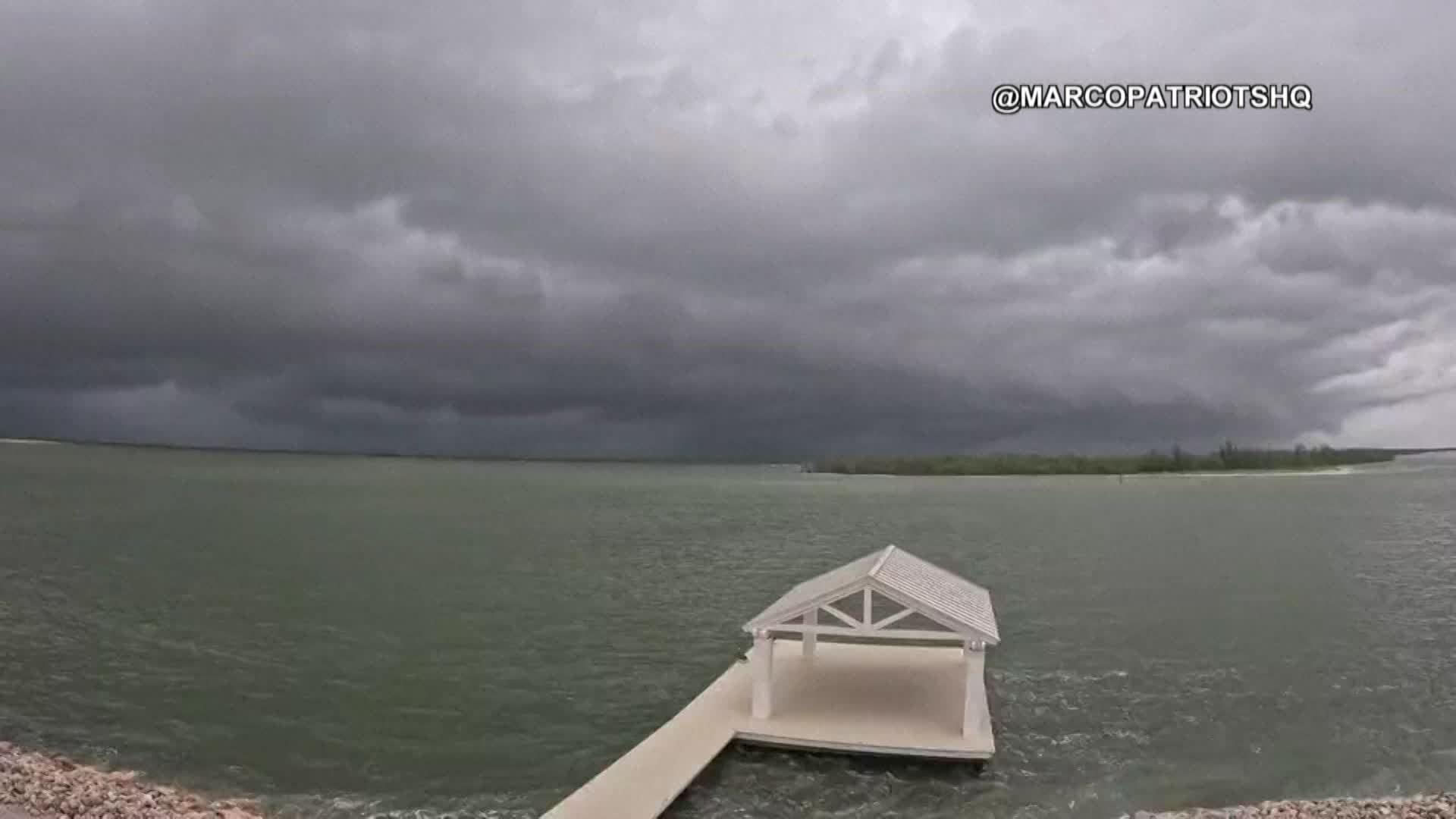A photograph, possibly a webcam image, captures a serene yet foreboding scene of a calm greenish lake on an extremely cloudy day. The vantage point is from the shore, where brown rocks line the bottom left corner. Extending into the lake is a long white pier leading to a covered dock with a white roof and pillars. The sky is dense with dark gray clouds, suggesting an impending storm. To the right in the distance, a tree-covered sandbar or small island is visible, adding to the scene's depth and complexity. The water exhibits slight ripples, hinting at the wind's effect, and overall, the image conveys a sense of calm before a storm. Noticeably, the scene is marked by “at Marco Patriots HQ” in the upper right corner, suggesting the location or source of the image.